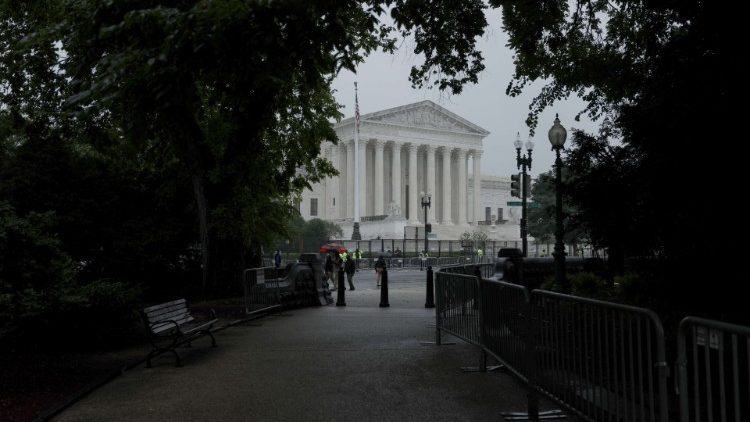The image captures the iconic Lincoln Memorial in Washington D.C., framed beautifully from within a park walkway. The main focus is the distinct white, columned building, with its eight grand columns and triangular pediment prominently jutting out. This memorial, which stretches its wings on both sides, is surrounded by a scenic park pathway lined with tall trees and lush greenery, creating a picturesque and serene setting. Along this walkway, one can also notice several benches inviting passersby to rest. A waist-high metal railing borders the pathway, directing foot traffic and adding to the organized layout of the surroundings. In the distance, near the memorial, individuals in high-visibility jackets, likely security personnel, can be seen near a black fence and shorter silver barriers that provide an added layer of security around the structure. Pedestrians meander along the wide, paved walkway that looks like a street but is restricted to foot traffic, further contributing to the lively yet ordered atmosphere of the scene.